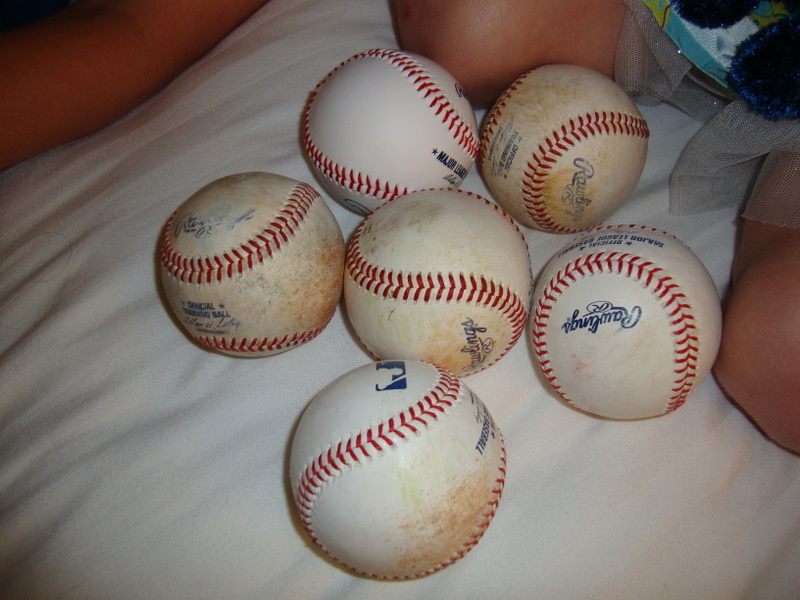The image captures six Rawlings baseballs placed on a soft, white surface, presumably a bed. In the forefront of the image, near the bottom, there appear to be the knees of a child kneeling on the bed. The baseballs, all featuring white covers with red stitching and blue Rawlings logos, vary in their condition. One baseball appears new and pristine, while two have minor mud stains. The remaining three baseballs are significantly dirtied and discolored with yellowish mud stains. In the background, there's a hint of clutter, possibly involving an arm or knee, and a bed frame is slightly visible at the back left of the image.